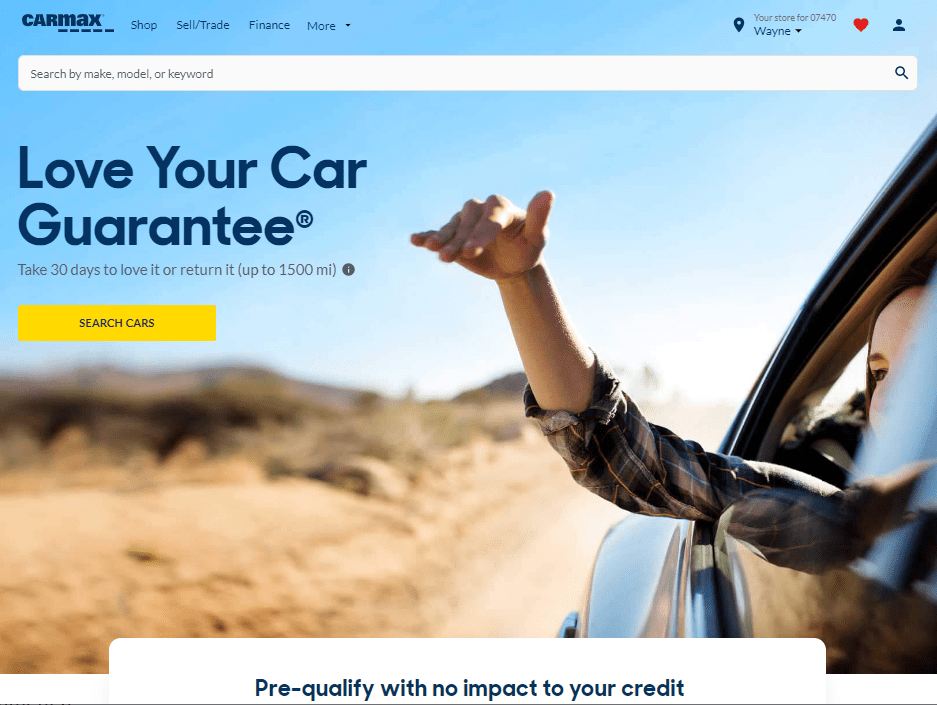A vibrant photograph from the CARMAX website showcases an engaging scene set against a predominantly blue sky that transitions to white near the horizon. Featured on the right side of the image is a passenger in a car, wearing a plaid shirt, with her hand extended out of the window. Her hand is playfully shaped like an airplane, surfing the wind, capturing a moment of carefree joy. Only the side of her face, including part of her eye and nose, is visible. The car appears to be driving along a road bordered by dirt, dry grass, and weeds, with distant hills adding depth to the scenery. Above this picturesque backdrop, the CARMAX website's interface includes a search bar prompting users to search by make, model, or keyword. Below this, in dark navy print, the text reads "Love Your Car Guarantee," followed by smaller text detailing, "Take 30 days to love it or return it up to 1500 miles." A prominent yellow button labeled "Search Cars" completes the user interface, encouraging visitors to begin their car search.